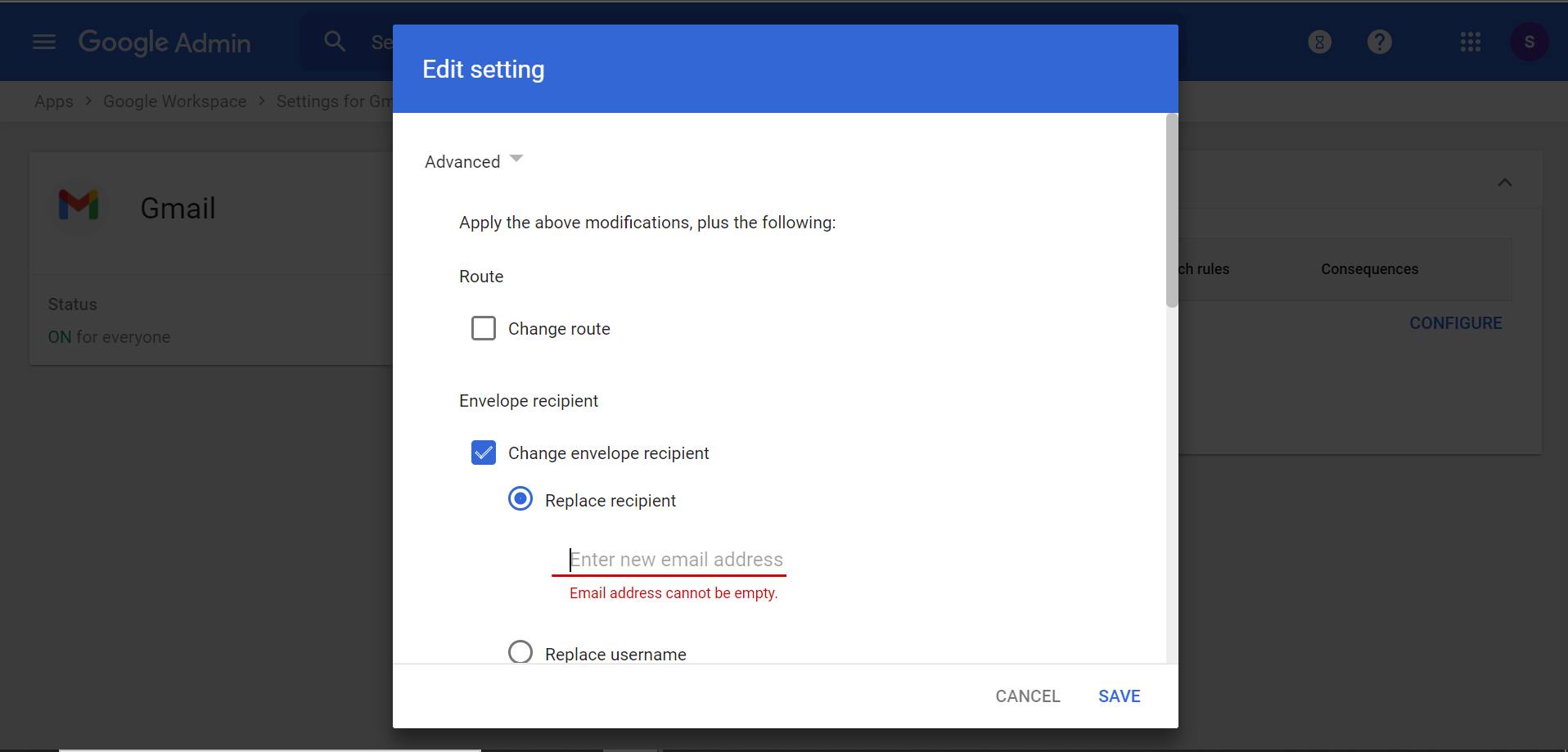The image is a screenshot from the Google Admin console. The primary focus of the screenshot is a pop-up box that overlays a grayed-out background of the Google Admin interface. On the upper left, the words "Google Admin" are faintly visible, and just below that, the Gmail logo – an envelope adorned with Google’s signature colors – appears alongside the text "Gmail."

Front and center is the prominent pop-up box with a white background and a blue header. The header reads "Edit Settings" in white text. Below that, on the left side, there's an "Advanced" label followed by an inverted triangle indicating a drop-down menu. Beneath this, it reads: "Apply the above modifications plus the following."

Further down, there are options such as "Root" and "Change Root," accompanied by a gray checkbox that can be selected. Next, the option "Envelope Recipient" is listed with "Change Envelope Recipient" below it. This latter option is checked, signified by a blue box with a white checkmark. Additionally, “Replace Recipient” is marked with a blue dot.

A red line follows, under which the text "Enter New Email Address" appears. In red text below that, it warns, "Email Address Cannot Be Empty." Lastly, the "Replace Username" option is displayed.

In the lower right-hand corner of the pop-up box, there are two buttons: "Save" and "Cancel."